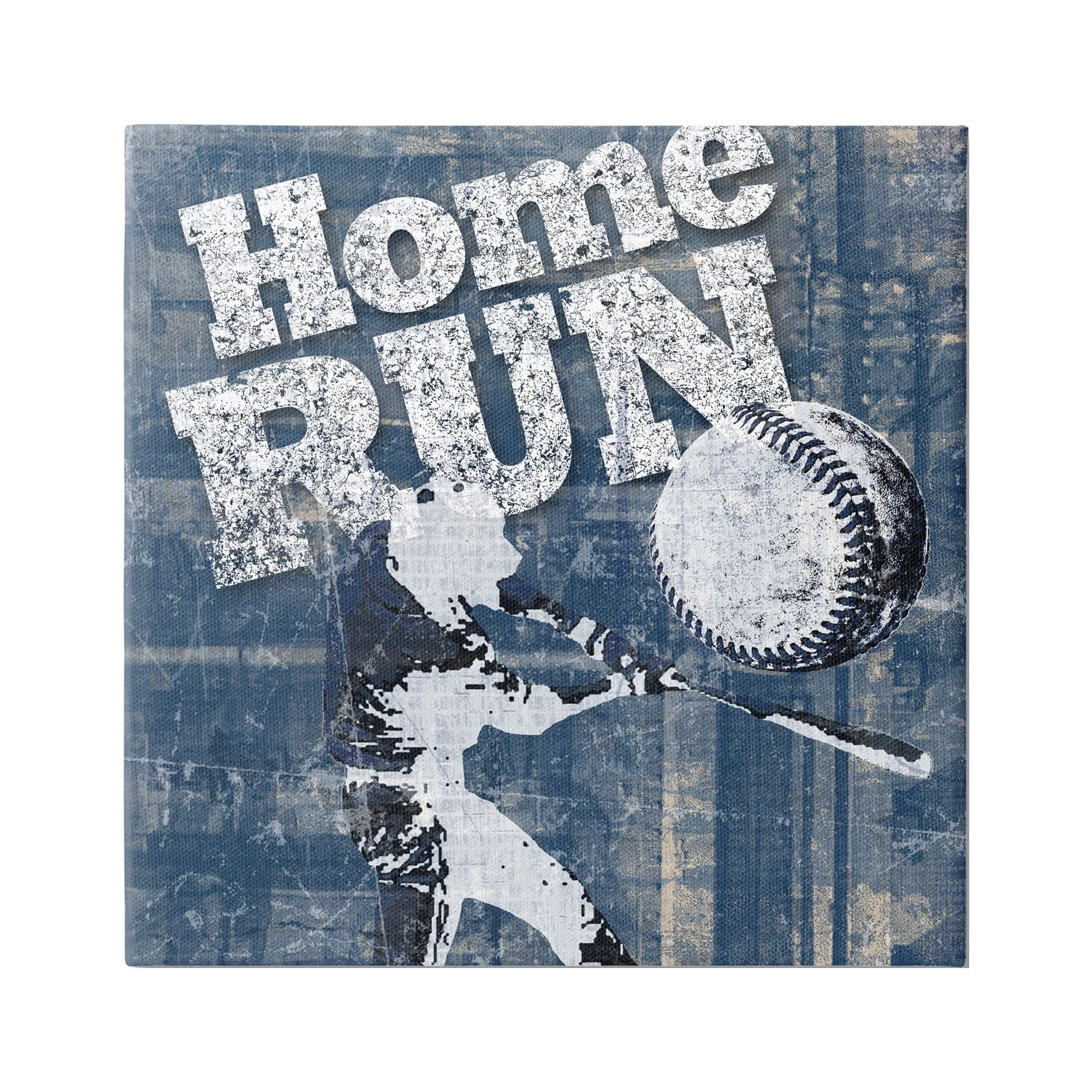The image depicts a distressed, navy blue square with a textured, worn appearance reminiscent of faded, torn jeans or denim. At the center, there's a large, round baseball rendered in white with detailed gray and black contours. Below it, in a sporty serif font, the words "Home Run" are stenciled in a faded white, enhancing the weathered and scratched-up look of the entire image.

A dynamic and abstract stencil of a baseball player swings a bat with significant might and power. The player is primarily depicted in shades of blue and white, with hints of black, and although his features are indistinct and somewhat animalistic, his stance conveys strong movement and energy. The overall aesthetic combines the vintage feel of the distressed background with the powerful imagery of the athlete in action, creating a visually striking representation.